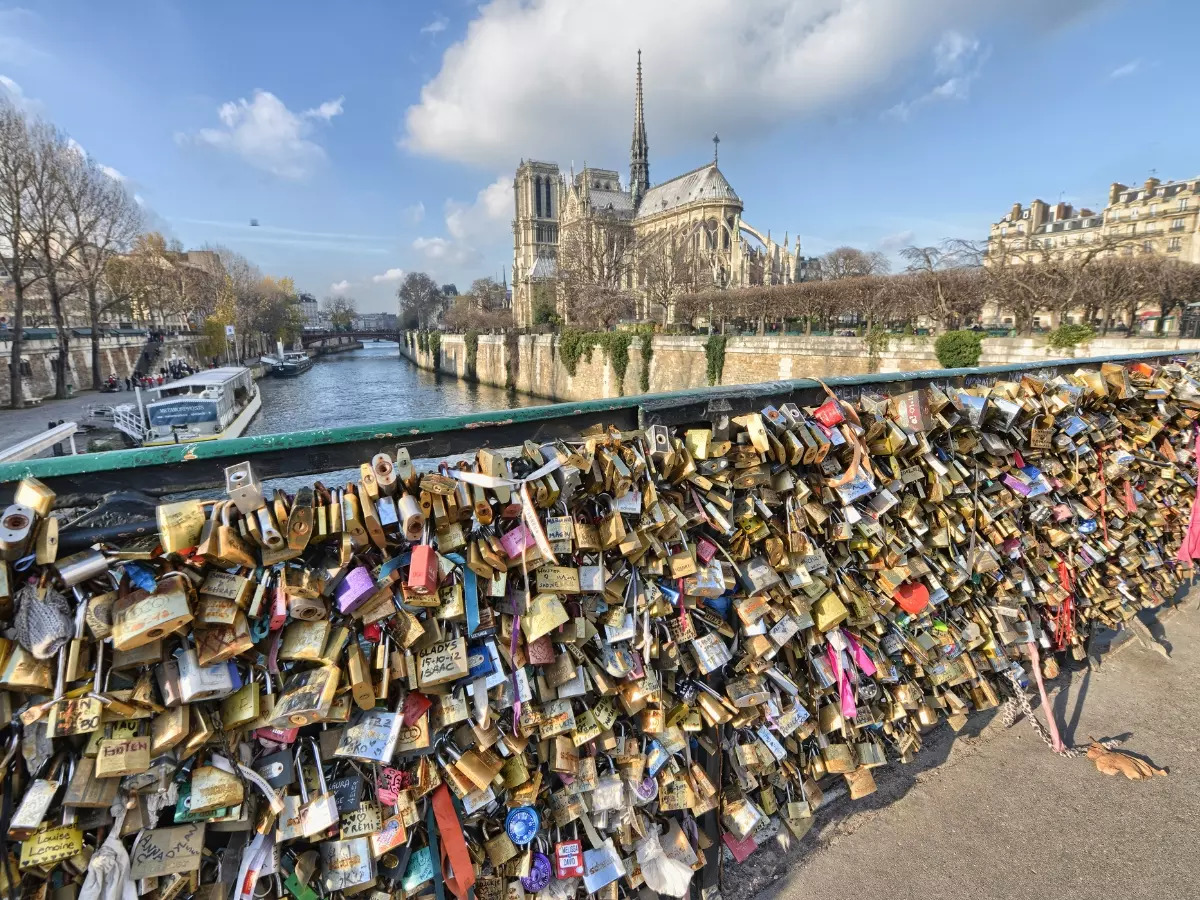The image depicts a bustling outdoor scene in a European city, notably with a vibrant blue sky accented by some clouds primarily in the center and to the left. On the left-hand side of the image, a line of trees stands tall with buildings nestled behind them. A concrete wall forms the boundary of a waterway that runs through the town, where several sizable boats are docked along its left-hand edge, creating a serene dockside ambiance. 

To the right, industrial buildings with a sense of aged charm rise up, juxtaposed with a palatial-style building in the background. Trees in this area appear somewhat barren at the top, contrasting with the lush greenery on the left. Center stage is a well-documented footbridge adorned with an array of locks in diverse colors – gold, brass, silver – and some decorated with vibrant ribbons. This common tradition, often symbolizing love, features locks marked with a multitude of handwritten names and texts. Notable names such as 'Gladys 151012 Isaac' are highlighted among the masses. 

The bridge, situated over what might be the River Seine in Paris near the Notre Dame Cathedral, becomes a focal point of cultural and historical significance. The sunlight reflecting off the locks creates a stunning golden sheen, adding to the picturesque quality of this sunny day.